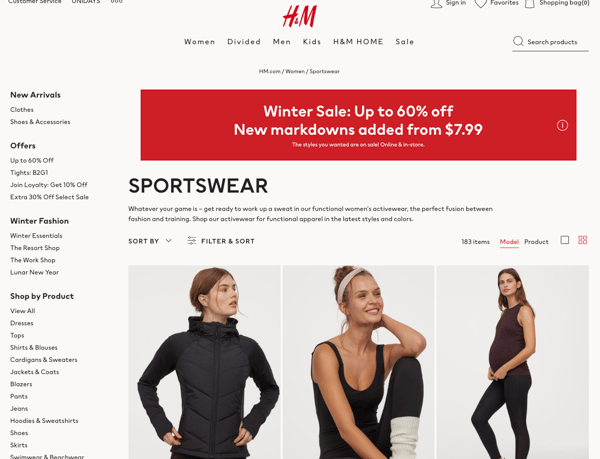The H&M website features a cream, off-white background. At the top, there's a prominent banner advertisement announcing a winter sale with discounts up to 60%, and new markdowns starting from $7.99. The website's main sections are clearly listed: Women, Divided, Men, Kids, H&M Home, Sale, and a search bar on the right, along with options to sign in, view favorites, and access the shopping bag.

On the left side, a menu categorizes clothing items into specifics such as dresses, tops, shirts and blouses, cardigans and sweaters, jackets and coats, blazers, pants, jeans, hoodies, and more. The featured section displays sportswear, showcasing three female models, all white women dressed in black athletic wear. 

One model appears to be pregnant, adorned in form-fitting leggings and a sleeveless shirt. Another model has a ballerina-like appearance, complete with rolled-up socks. The model on the left is pictured in a snug raincoat. The sportswear section emphasizes a blend of function and style, catering to diverse athletic and casual wear needs.